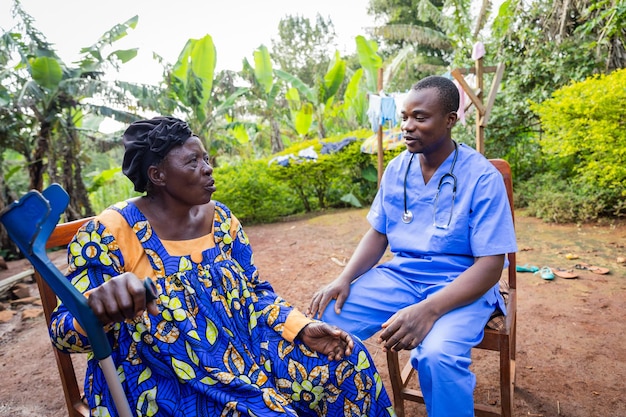In this detailed photograph, two people are sitting in wooden chairs in a cleared dirt area amidst a lush, tropical environment. The background is teeming with green hedges, palm trees, and other dense vegetation, giving the impression of a jungle or tropical forest clearing. Pairs of sandals are scattered on the ground, and a clothesline with various garments hangs to dry in the background.

On the left side of the image, an older black woman, likely in her 60s, is seated. She wears a vivid blue mumu adorned with green floral and leaf patterns, under which an orange shirt is visible. Her hair is concealed by a black turban or head wrap. The woman appears to be mid-conversation, captured with one hand grasping a crutch for support, and her expression hints at concern or anxiety.

To her right is a younger black man, probably in his late 20s to early 30s, dressed in blue hospital scrubs with a stethoscope draped around his neck, suggesting he is a doctor or medical professional. He sits in a relaxed manner, also engaged in the conversation, with a warm, reassuring smile. The interaction between them seems to be a medical consultation or discussion, taking place outdoors in daylight. The serene yet attentive demeanor of the man contrasts with the woman's worried look, hinting at a compassionate exchange amidst a vibrant natural setting.